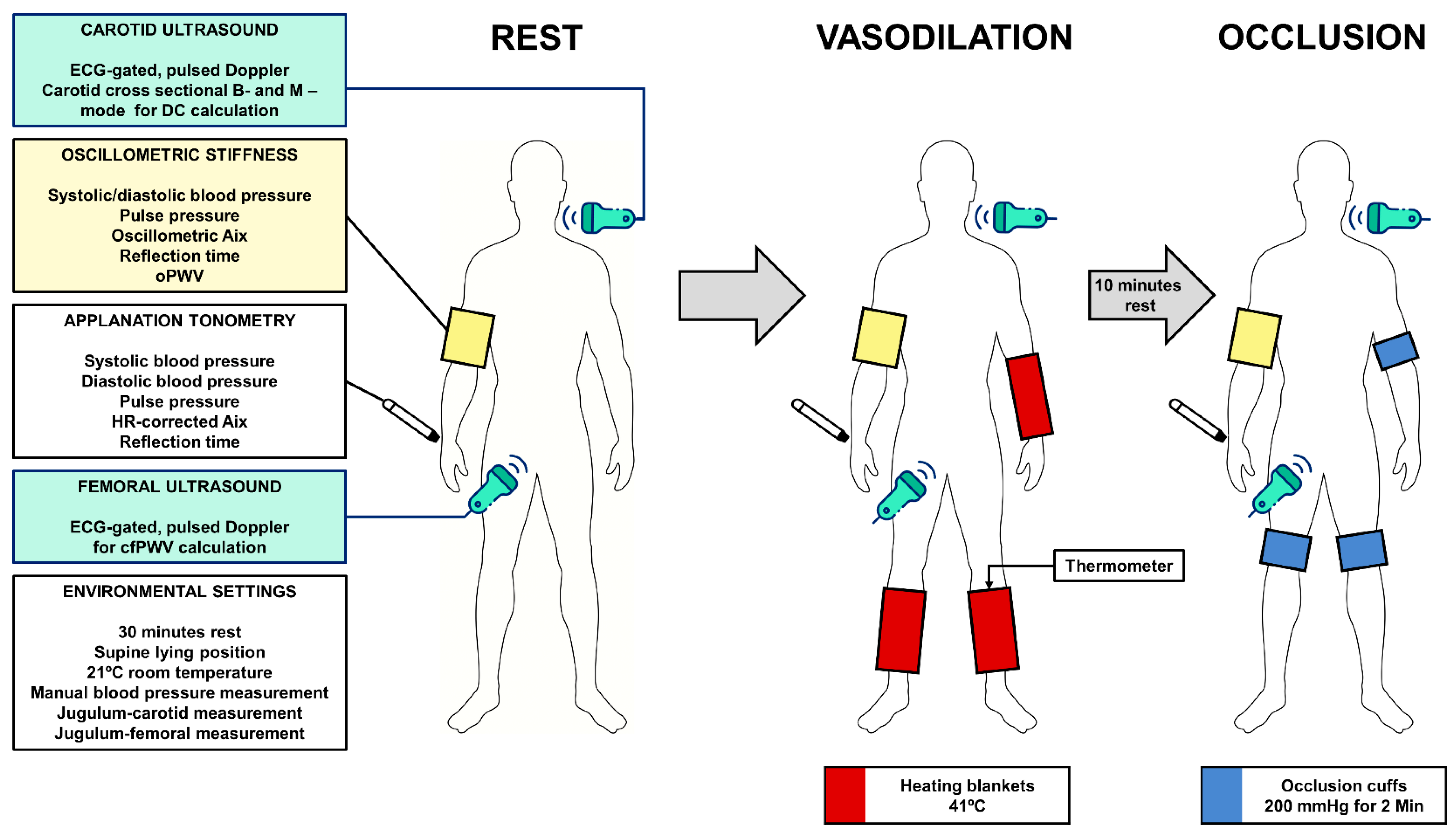This detailed medical flowchart illustration showcases three identical human figures each labeled "Rest," "Vasodilation," and "Occlusion." The entire diagram is set against a white background. The "Rest" figure displays various medical instruments and measurements: a green device pointed at the neck connects via a line to a box labeled "Carotid Ultrasound, ECG gated, pulsed Doppler, carotid cross-sectional B- and M-mode for DC calculation." Another instrument points to the right elbow with a yellow band, leading to a box labeled "Oscillometric stiffness, systolic, diastolic blood pressure, pulse pressure, oscillometric AIX reflection time, OPWV." Additionally, a rod aims at the right wrist, connecting to "Applanation tonometry, systolic blood pressure, diastolic blood pressure, pulse pressure, HR corrected AIX reflection time." A green device near the crotch links to "Femoral ultrasound, ECG gated, pulsed Doppler for CFPWV calculation." This section also specifies "Environmental settings: 30 minutes rest in a supine position at 21 degrees Celsius, manual blood pressure measurement, jugular carotid measurement, and jugular femoral measurement."

The "Vasodilation" figure includes similar technical details with green instruments at the ear and crotch, and a rod at the wrist, but also features heating blankets indicated by bands on the right arm and both shins, set to 41 degrees Celsius, following a 10-minute rest period.

Lastly, the "Occlusion" figure depicts the same green instruments and attachments with an added yellow band above the right bicep, a blue band at the elbow, and blue bands on the knees, indicating the use of occlusion cuffs set to 200 mm Hg for 2 minutes.